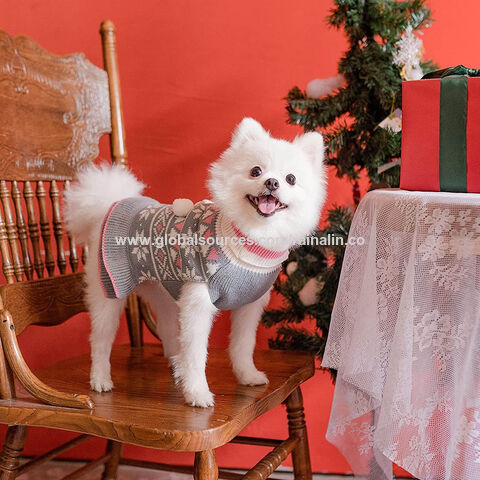In this charming holiday scene, a small, fluffy white dog stands proudly on an old-style wooden railback kitchen chair. The dog is wearing a festive Christmas sweater with a gray background adorned with a Nordic print in white, red, and green, featuring snowflakes. His round black eyes and small black nose peek out as he turns his head towards the camera, giving the impression of a joyful smile. To the right of the dog, a table draped in a white cloth with floral and leaf patterns holds a beautifully wrapped red Christmas present with a green ribbon and bow. The background features a decorated Christmas tree, seemingly artificial with hints of faux snow on its branches. The wall behind the scene is a warm orangish-red hue, adding to the cozy holiday atmosphere. The image also contains partially visible white text over the dog that starts with "www.globalsourses" and ends with "n-a-l-i-n dot co," obscured where it overlaps with the dog's fur. The floor beneath the scene appears to be white or gray, completing this festive snapshot.